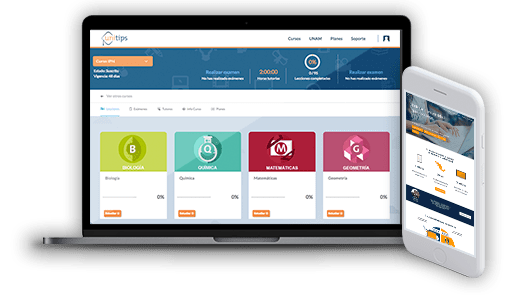A high-resolution product image showcases the UniTips application displayed on both a laptop and a white cell phone, emphasizing its cross-platform functionality. On the laptop screen, the UniTips interface features a lineup of colored rectangular icons stretching across the display. From left to right, each icon is distinctively colored and labeled with a letter: a yellow 'B', a teal 'Q', a red 'M', and a dark pink 'G'. Despite the blur obscuring the text inside these boxes, the vibrant icons suggest a visually engaging and user-friendly design. The white phone positioned to the right of the laptop further underscores the application's compatibility with multiple devices, making UniTips a versatile tool for various users.